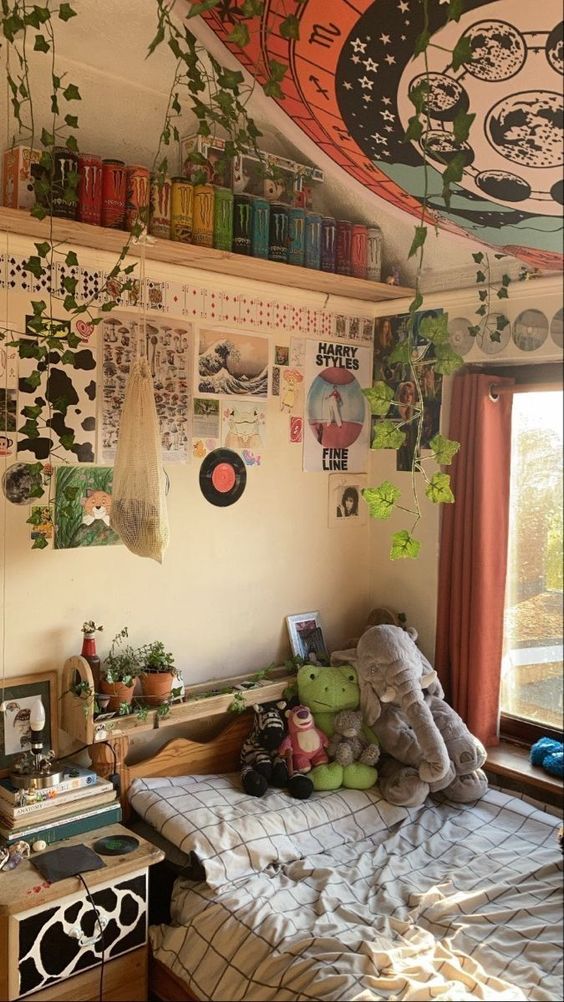The photograph captures a cozy, well-decorated kid's bedroom with vibrant and detailed elements giving it a personalized touch. The centerpiece is a small bed with crumpled checkered sheets predominantly featuring white squares outlined by black lines. The bed is adorned with an assortment of stuffed toys, including an elephant, a frog, a zebra, and a small bear that resembles the character from Toy Story 3. To the left of the bed stands a table or shelf holding an eclectic mix of objects, including a stack of books, a CD, and various other items.

Above the table, a variety of objects rest on a shelf, most notably a line of colorful Monster Energy drink cans forming a rainbow array, with approximately 15 cans positioned upright. The wall behind the bed is decorated with posters, including one of Harry Styles, a circular LP record sticker with a distinctive red center, and a row of playing cards. Hanging from the ceiling, green leafy vines add a touch of nature, complementing the scattered plants and flowerpots throughout the room.

A prominent window to the right, framed by red curtains, allows natural light to filter into the space. The ceiling features a tapestry displaying the phases of the moon, contributing to the room's whimsical and slightly mystical ambiance. The overall setting suggests a top-floor location with an angled ceiling, adding to the room's unique character. Despite its cozy appearance, the bed doesn’t seem exceptionally comfortable, but the personal touches and vibrant decorations certainly make it a charming and inviting space for a child.